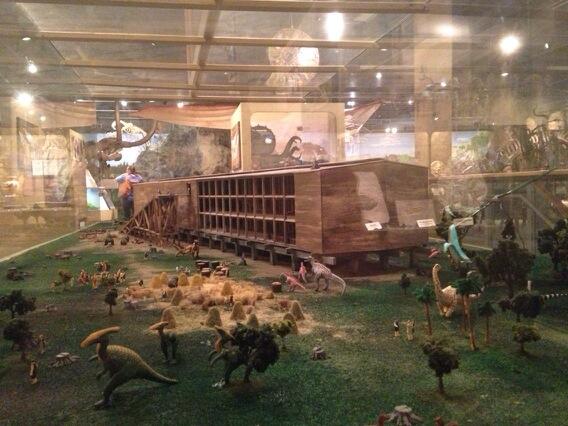The image portrays a detailed miniature model displayed inside a glass case situated within a well-lit indoor space, likely a museum. The model features a large, green grassy field dotted with several trees and small piles of hay. Dominating the center of the scene is a massive, three-level wooden structure resembling the construction of Noah's Ark, with multiple square openings on each level and a flat roof. Surrounding this structure, one can see an assortment of small, colorful dinosaur figurines—some green, yellow, and red—scattered across the field. In the background of the larger room, which is partially obscured, there are various bins and containers and a person with a bag on their shoulder, suggesting additional exhibits or storage typical of a museum environment.